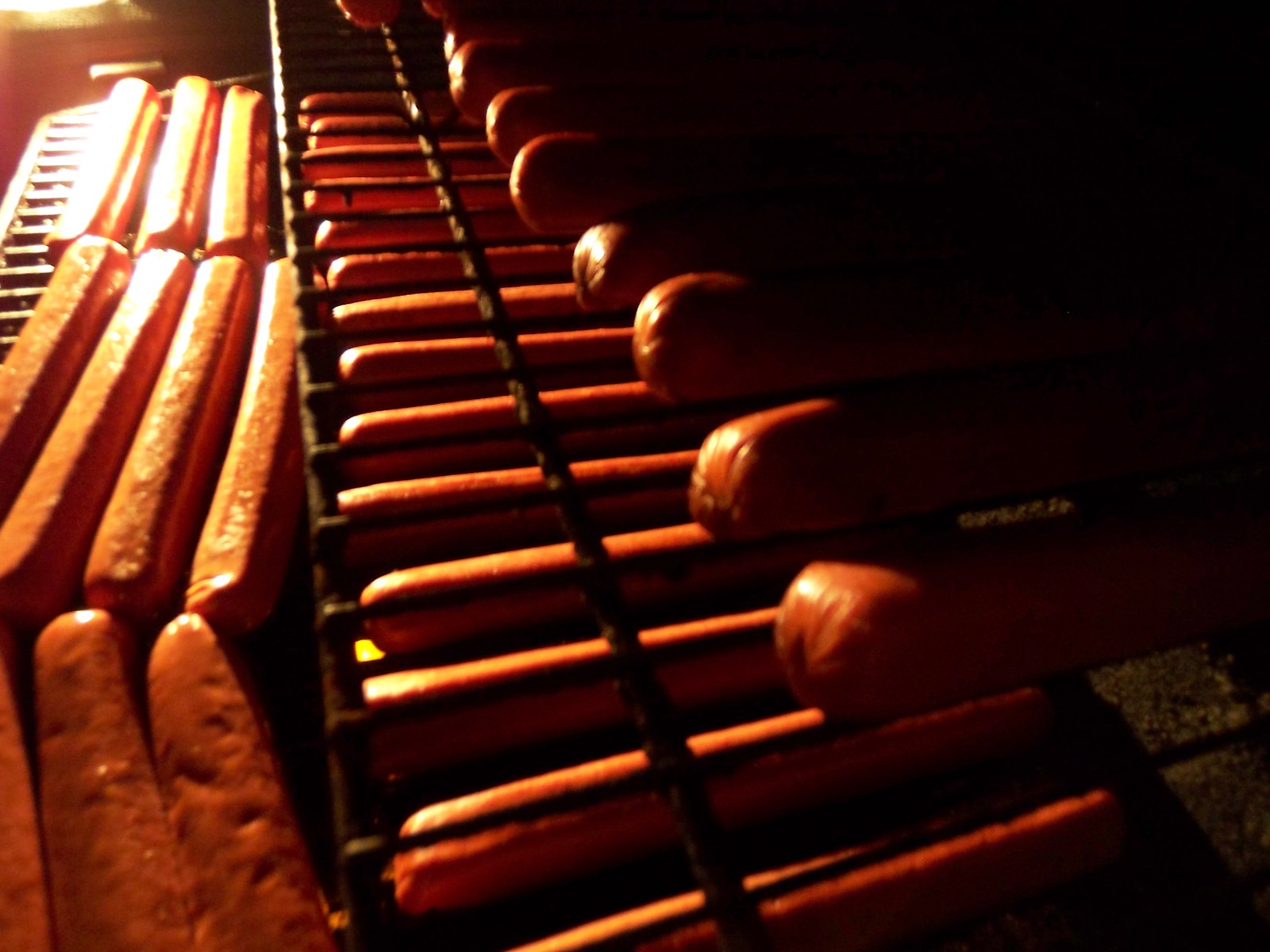This photograph captures an artistically styled scene of numerous uncooked hot dogs meticulously lined up on a large, black commercial grill. The grill doesn't appear to be fired on yet, as no glowing coals are visible. The hot dogs, numbered at least two dozen, are arranged in orderly rows, both horizontally and vertically, covering the grill's surface. Among the uniform reddish-pink hot dogs, one stands out with noticeable dimples. Notably, the grill seems to be a double-tiered system, with more hot dogs visible through the grates below the top layer, indicating a setup meant for mass cooking rather than a backyard barbeque. The photograph is dark and high-contrast, with the lighting casting shadows from the upper left, adding depth and a dramatic effect to the image.